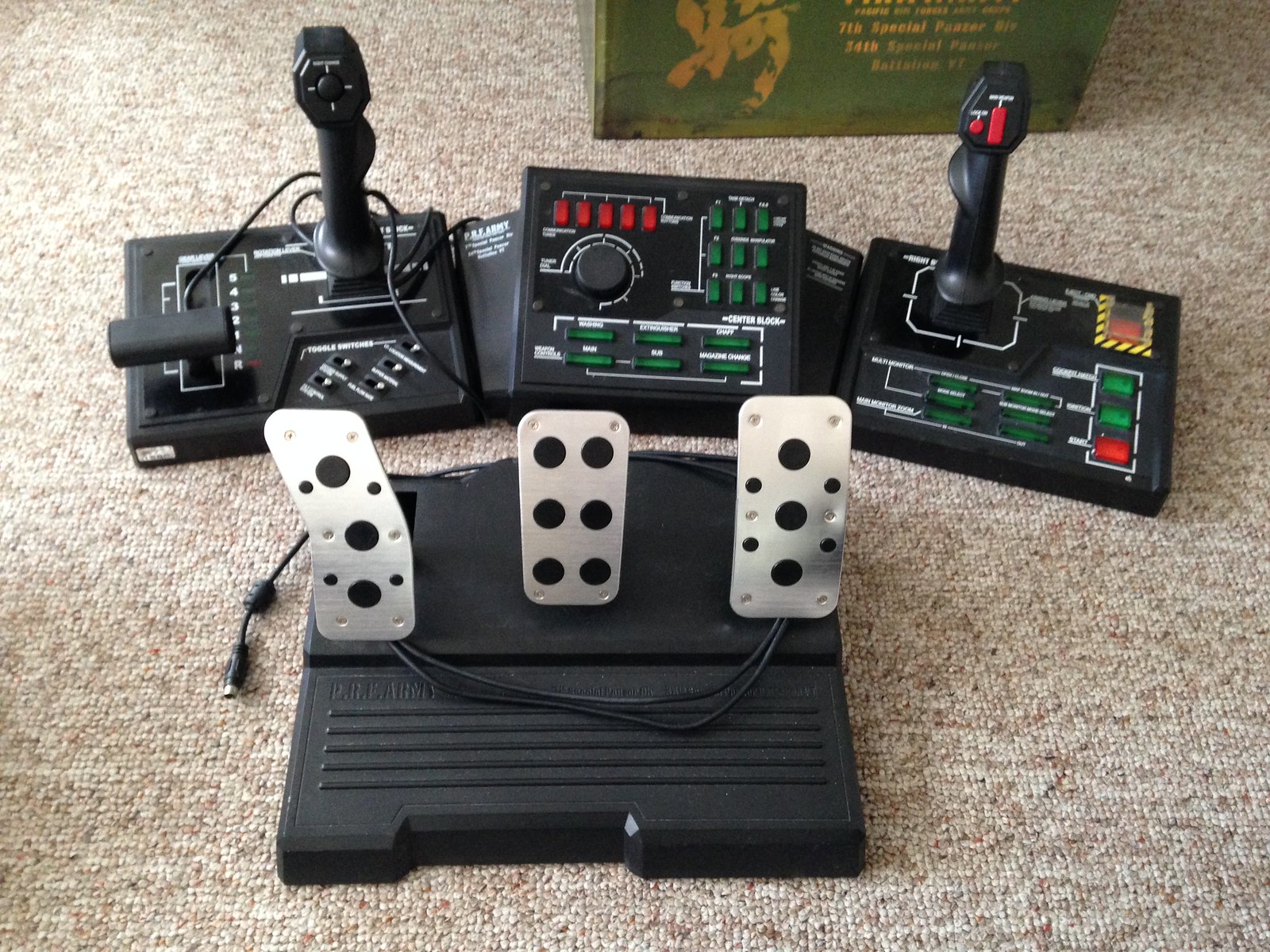This overhead photograph showcases a sophisticated gaming setup on a tan, Berber-style carpet. Central to the image is a black console equipped with two joysticks, foot pedals, and an array of control buttons. The pedals are housed in a robust black base and consist of three silver elements: the brake, the clutch, and the gas pedal. Distinctively, each pedal features medium-sized black dots for traction—three on both the brake and the gas, and six on the clutch.

Positioned on the left wing of the console is a joystick with black control buttons, complemented by a gear shift labeled with positions 1 through 5, neutral, and reverse. The right wing holds a joystick adorned with red buttons. Nestled between the joysticks, the console brims with additional controls, including hunter green and red buttons. A prominent feature is a black knob encircled by a white dial, potentially for adjusting settings. An emergency off switch, marked conspicuously by a yellow and black roadway sign pattern, adds a safety element to the device. The entire setup is connected via cords leading to a computer, emphasizing its functionality for high-end simulations or gaming experiences.